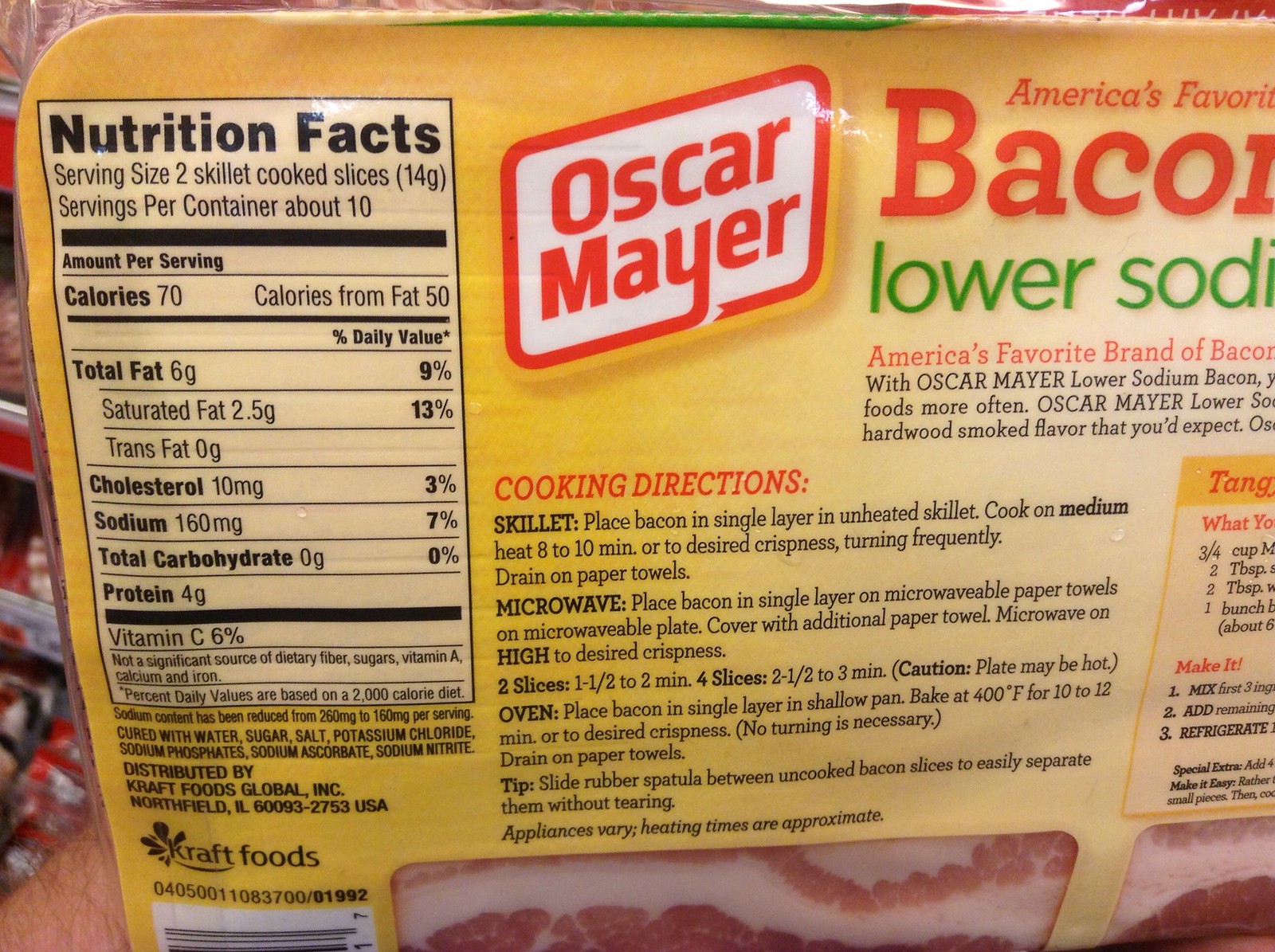This image, in landscape format, depicts the back of an unopened Oscar Mayer bacon packet. The package is primarily yellow with a clear plastic section at the bottom, revealing the pink and white bacon inside. On the upper left, nutrition facts are prominently displayed, and directly below that are the ingredients. The Oscar Mayer logo, a white background with red text bordered by a thin red line, is located near the top. Adjacent to the logo are the words "America's Favorite Bacon" and "Lower Sodium," written in green and red. Beneath this text, cooking directions for skillet, microwave, and oven methods are detailed. In the lower left corner, the packaging mentions Kraft Foods. Some transparent holes near the bottom provide a glimpse of the neatly lined bacon slices, highlighting its meaty and fatty texture. This detailed presentation of the Oscar Mayer bacon package is typical for grocery store aisles.